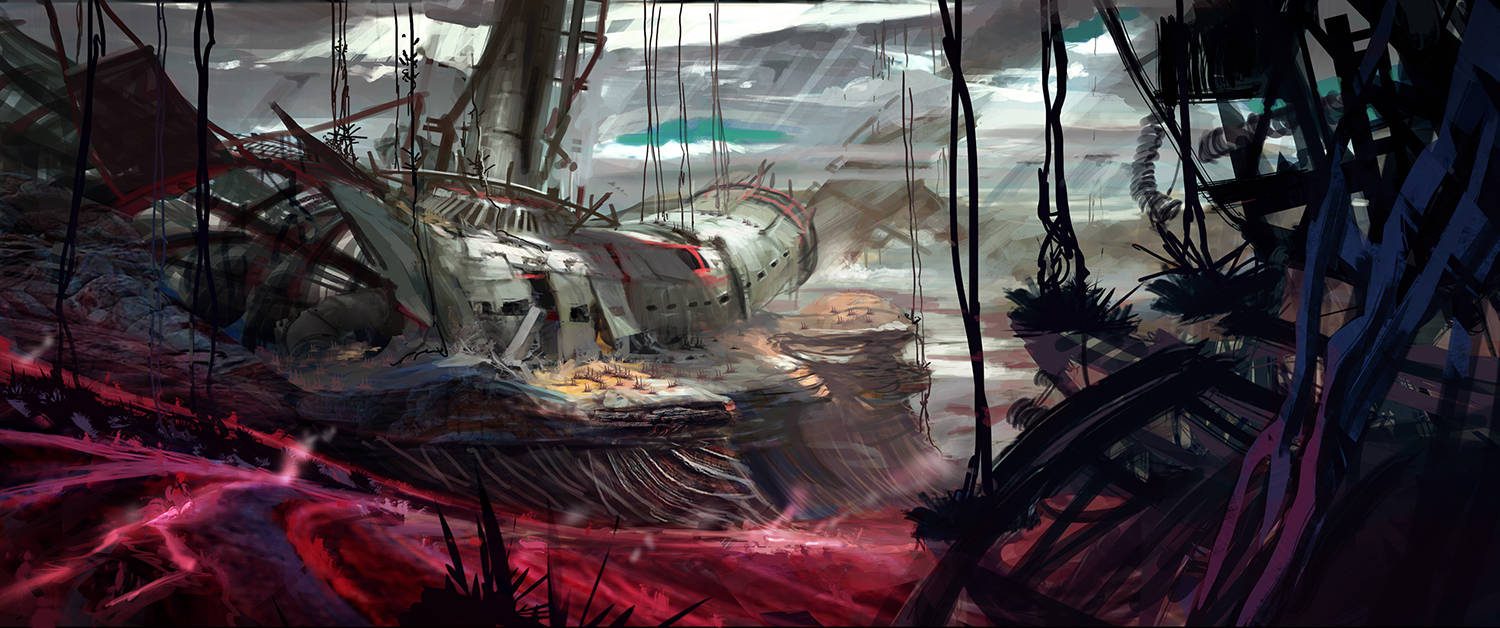This AI-generated, highly stylized image depicts a dramatic, eerie scene of a heavily damaged, sunken or crashed ship that might also be a destroyed spaceship, laying on a brown, tree-root-supported plateau, possibly underwater or in another murky environment. The ship is positioned on its side, predominantly colored in gray with red accents, and features a conspicuous tower protruding from the top. The ambiance is emphasized by distinct beams of light slicing through the murkiness, illuminating areas while most of the scene remains shadowy and obscure. The foreground is striking with hues of red and a potential fiery or lava-like presence, contrasting against a dark and predominantly grayish background. Vines or cables hang down from above, partially obscuring the view and adding to the sense of decay and abandonment. Amid the darkness and desolation, the upper left section displays what appears to be a flag, contributing to the overall somber and ominous atmosphere.